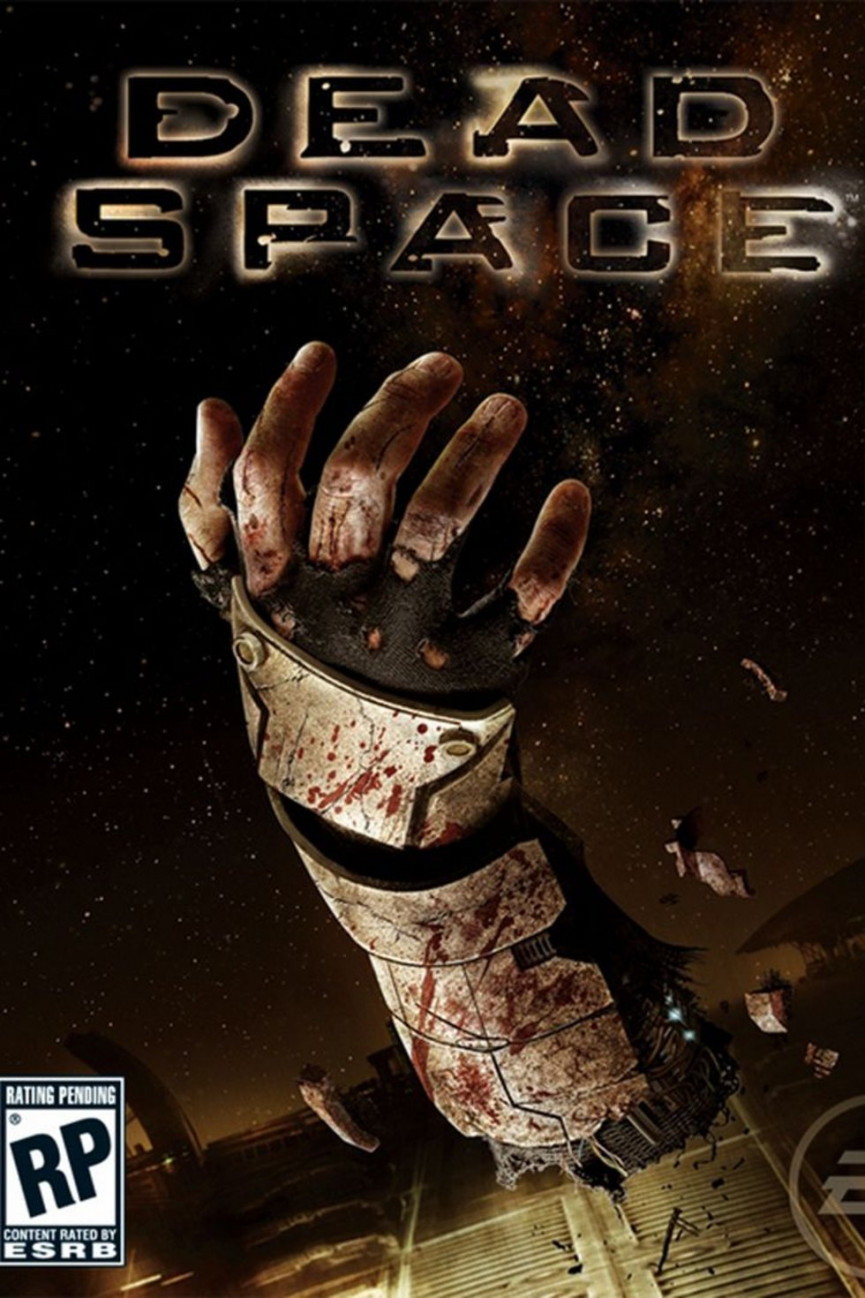This is the cover of the video game "Dead Space." The primary focus is a large, dismembered right hand and wrist, suspended in space, with visible scrapes and blood. The hand, clad in black and gold armor, appears to have been brutally severed. The dark sky forms the background with scattered stars, creating an ominous atmosphere. The title "Dead Space" is prominently displayed in bold, white-lit, uppercase letters at the top of the image. At the bottom left corner, a black-and-white rectangle holds the "Rating Pending" (RP) symbol, indicating the game has not yet been rated, along with "Content Rated by ESRB" text. Additional details, such as pieces of space equipment and objects appearing to fall, are scattered at the bottom, enhancing the eerie, chaotic scene.